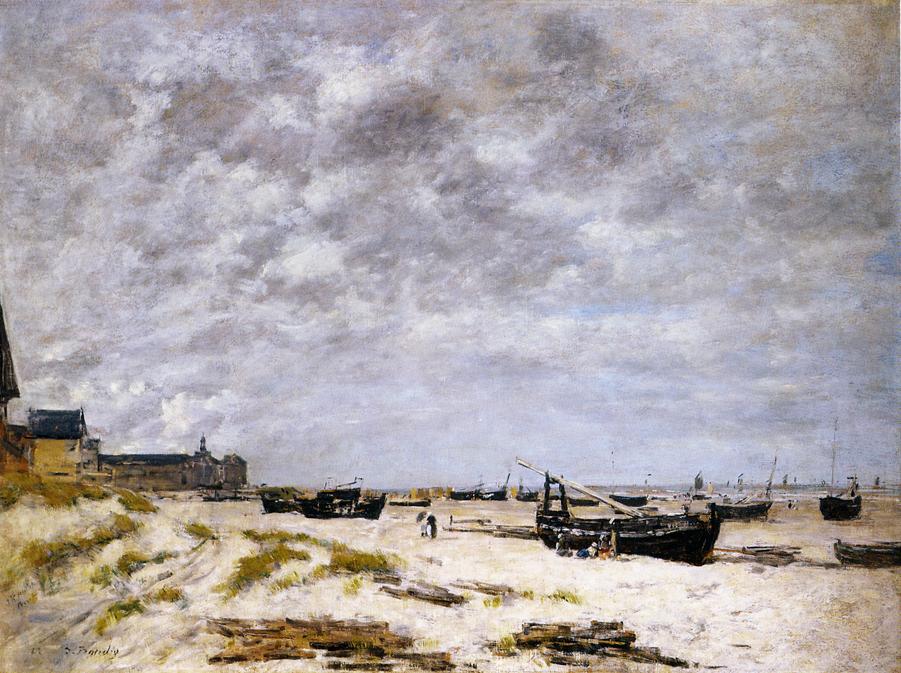This image captures a vivid seaside painting featuring a dynamic interplay of land, sea, and sky. The top portion is dominated by a dramatic sky filled with puffy white and grey clouds, giving an impression of an overcast day. As the clouds approach the horizon, they break up, revealing patches of darker blue sky, suggesting a mix of weather conditions. Below, the beach scene unfolds in detail: the sandy shore is dotted with several wooden boats, some ash-colored and appearing abandoned or stranded, waiting for the tide to return. A few figures walk along the beach, contributing to the painting's lively yet tranquil atmosphere. On the far left, there are indistinct buildings rendered in a slightly impressionistic style, with at least two homes - one brown and one bright yellow - standing out. These homes are nestled among dunes covered in green grasses, offering a natural barrier. Further out to sea, about a half dozen boats with raised sails dot the horizon, adding depth and a sense of ongoing activity to this charming coastal scene.